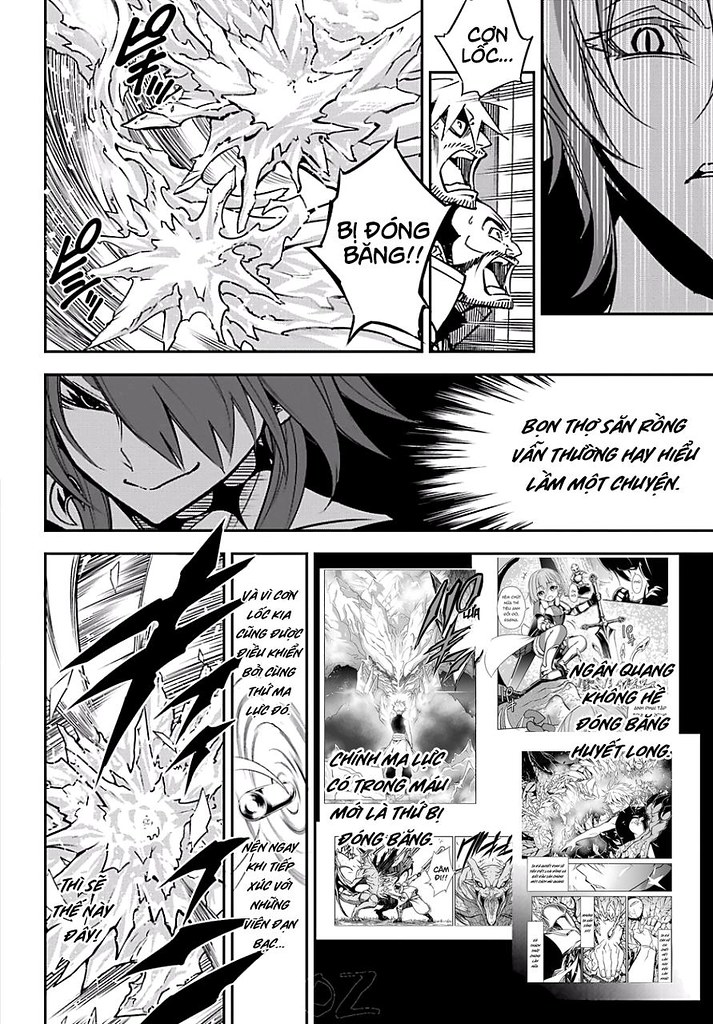The image resembles a black-and-white comic book page, possibly written in Taiwanese judging by the distinct lettering. The layout features several insets. In the center, there are two faces emerging from what seems to be violent waves or vapor, both in a distressful yell. Above this, a close-up of a person's terrified face dominates its panel. Just below, another face with a more devious, cunning expression is depicted. The bottom of the page contains four smaller, indistinct drawings, also bordered by the same mysterious water or vapor element found on the outside edges. This comic book-style artwork appears to be part of a larger narrative, filled with intense and dramatic moments.